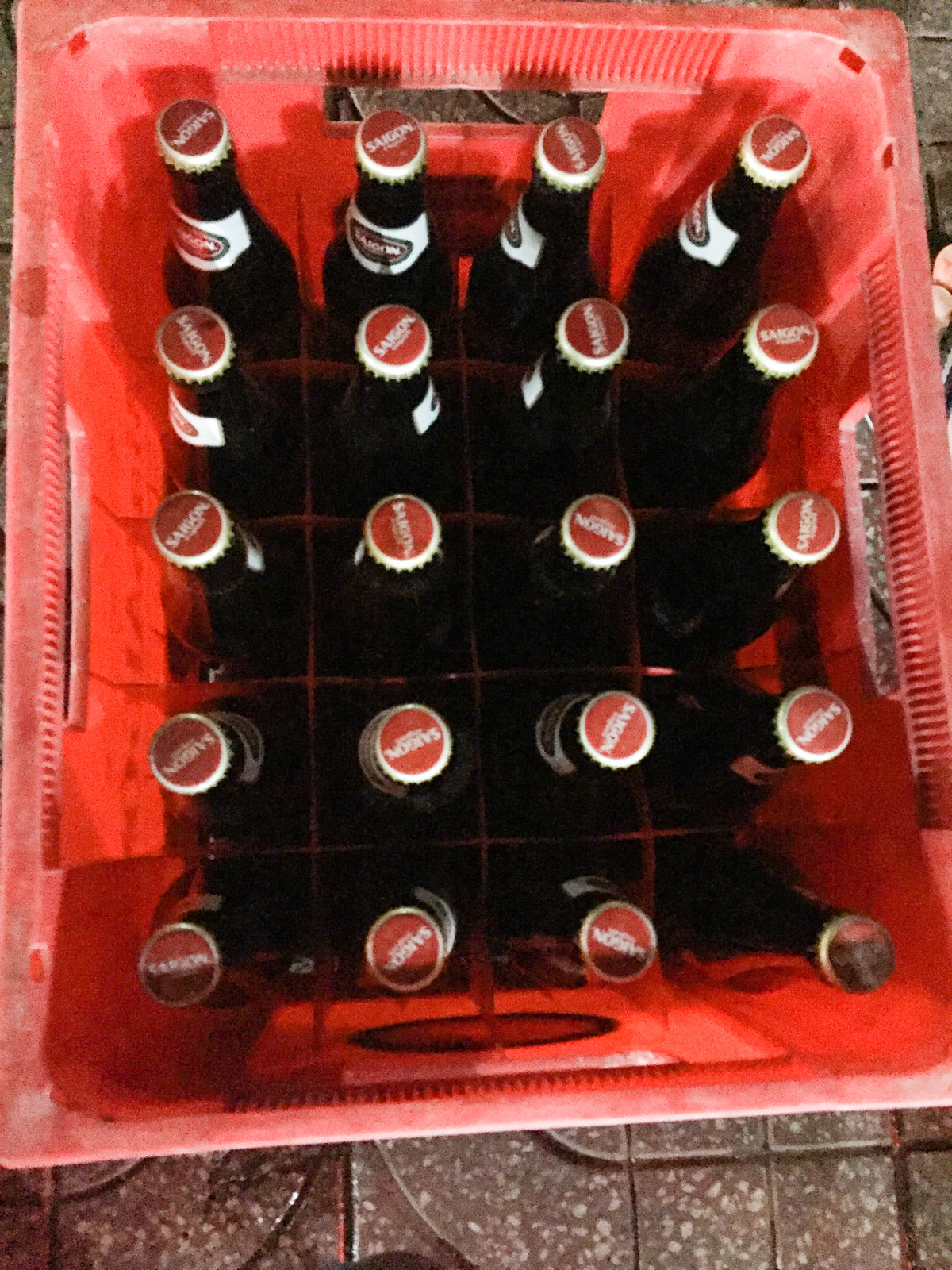This detailed aerial view photograph captures a faded red plastic crate housing twenty long-necked bottles, each capped with rigid, grooved metal caps. The bottles, with the brand name "Sasson" on the caps, might contain beer or a similar beverage, possibly soda. The crate, featuring a robust construction, is positioned on a cement floor that appears patterned but is only partially visible. The composition shows the bottles arranged neatly in four columns and five rows, emphasizing the orderly storage within the crate.